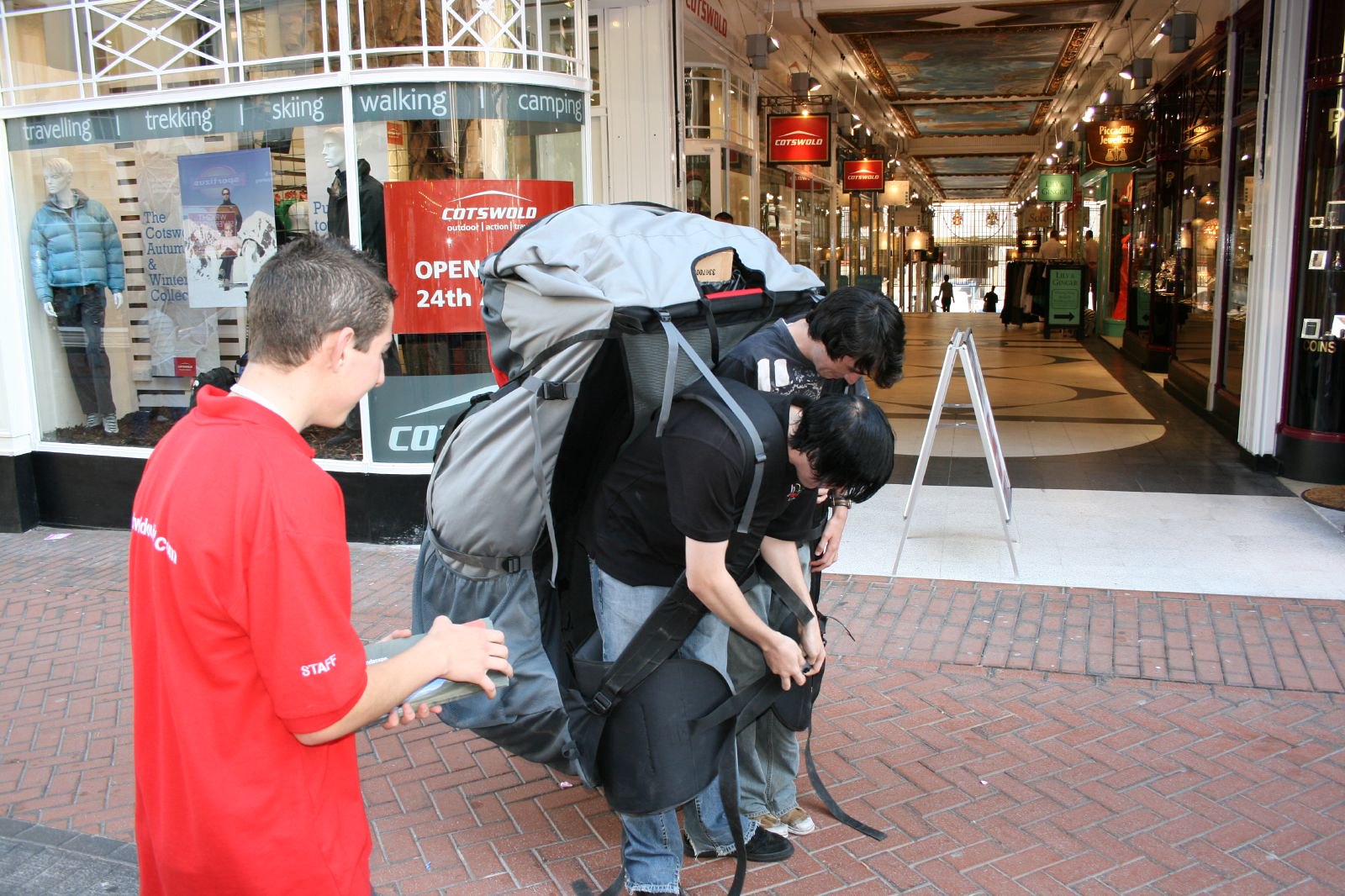This image is a realistic photograph, oriented as a horizontal rectangle, seemingly captured in an outdoor or possibly indoor shopping arcade. The ground consists of red bricks laid in a herringbone pattern. In the foreground, slightly to the left, stands a young, light-skinned male with short black hair, wearing a large red button-down shirt that says "staff" on the right sleeve. He appears to be laughing or observing something while holding a book or an object in his hands.

In the middle of the image, two males with dark hair, dressed in black t-shirts and blue jeans, are seen bending over, appearing strained as they carry an enormous, oversized gray backpack between them. This massive pack seems so heavy that it forces them to hunch. The two are teamed up, each strapped to the pack, navigating its weight together.

In the background, there is a glass-fronted store with signage that reads "Traveling, Trekking, Skiing, Walking, Camping." Additional store details include a mannequin dressed in a puffy blue jacket and black pants, a poster featuring a skiing scene, and a red sign that partially reads "Cotswold Open 24th."

The scene extends into a hallway with stores on either side, topped with an intricately designed ceiling featuring gold and green decor. The overall setting, with its ornate ceiling and ample lighting, suggests a bustling, fancy shopping area.